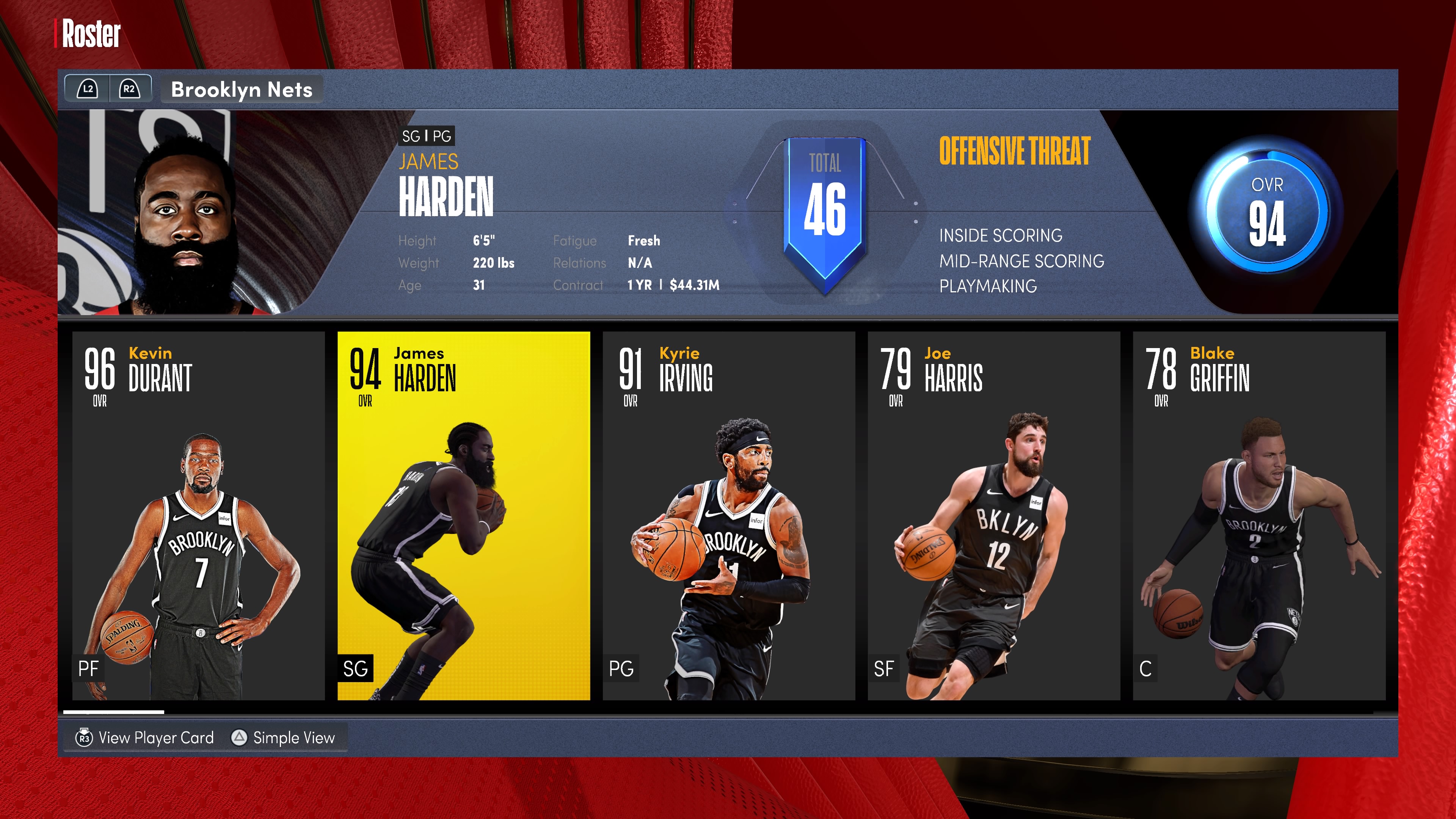The image features a vibrant red background that appears to resemble a curtain. In the top left corner, the word "Roster" is prominently displayed in white text. Just beneath this is a gray rectangular area, also in the top left corner in white text, stating "Brooklyn Nets." 

Directly below, the card presents a visual and textual profile of a basketball player. It depicts an African American man with a notably thick beard, identified as "James Harden." The text further details his physical attributes: height 6'3", weight 220 pounds, and age 31. Below these details, a blue ribbon indicates a "total" score of 46 and labels him an "Offensive Threat" with skills in inside scoring, mid-range scoring, and playmaking highlighted.

Lower on the image, there are five boxes. The first box on the left showcases "96 Kevin Durant," displaying an African American man clad in a black and white Brooklyn Nets jersey numbered 7. He is seen holding a basketball with one arm. To the right, a yellow-highlighted box shows "94 James Harden" once again, depicting him playing basketball and bending down, seemingly poised to take a shot.